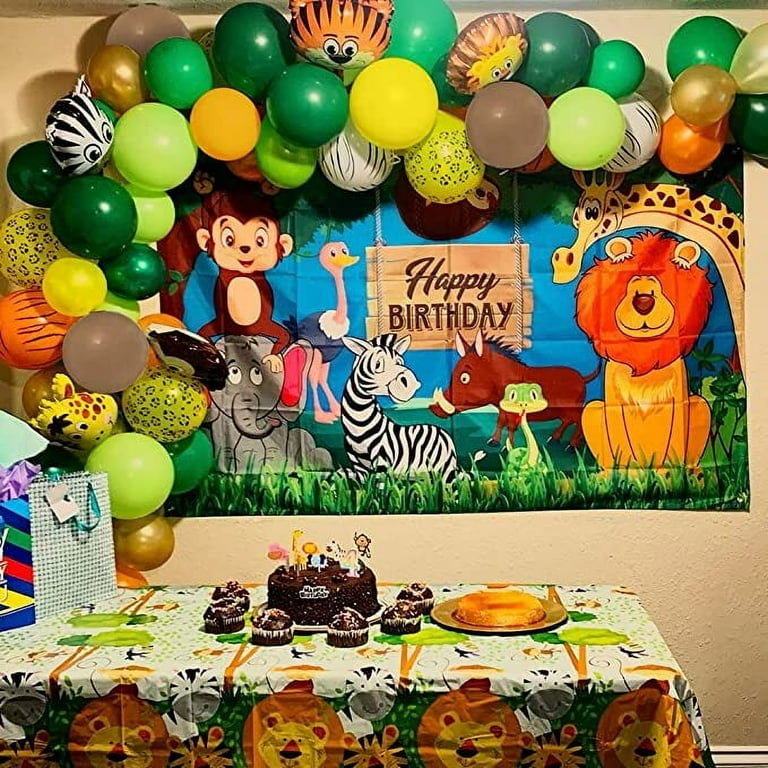This cheerful child's birthday party scene features a vibrant setup centered around a jungle and zoo animals theme. The backdrop showcases a large, bright-colored "Happy Birthday" banner adorned with playful cartoon animals, including a monkey perched on an elephant's head, an ostrich, an elephant, a zebra, a warthog, a snake, a grinning lion, and a giraffe. Surrounding the banner are an array of colorful balloons in primary colors such as green, yellow, and orange, complemented by mylar balloons in zebra, giraffe, tiger, and lion patterns.

In front of the banner, a table is covered with a matching, zoo-themed tablecloth featuring lions, zebras, and monkeys swinging through trees. The table is laden with festive treats, including a chocolate cake topped with jungle animal decorations like a monkey, giraffe, zebra, and lion, as well as a number four candle, indicating the age of the birthday child. Alongside the cake, there appear to be cupcakes or muffins, adding to the celebratory spread. To the left of the table are brightly decorated gift bags, enhancing the joyful and lively atmosphere of the party.